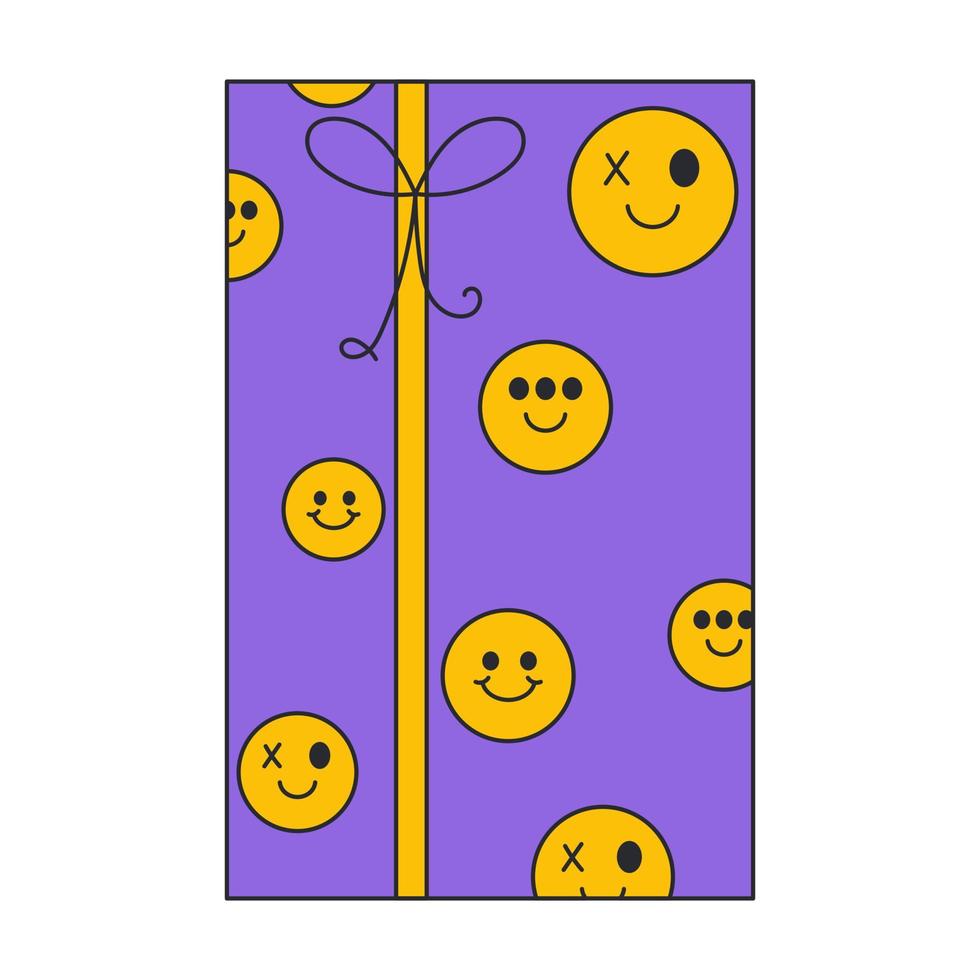The image is a rectangular illustration, approximately five inches high and three inches wide, set against a plain white backdrop. It features a thin black border that frames the image. The primary background color of the rectangle is purple. A vertical stripe in a gold or yellow gold hue, about three-quarters of an inch to an inch wide, runs from the top to the bottom along the upper left-hand side. This stripe is bordered by thin black lines on both sides. At the top of the stripe, a black pinstripe ribbon forms a bow, extending down about an inch.

Dominating the rest of the purple background are numerous yellow circular smiley faces with black outlines. The faces vary in size, with some displaying conventional designs of two eyes and a smiling mouth, while others are more whimsical: some smiley faces have three eyes, and others feature one eye depicted as a black oval while the other is a black X. The rich interplay of purple, yellow, and black imparts a playful and dynamic visual effect, suggesting an engaging graphic design or whimsical illustration.